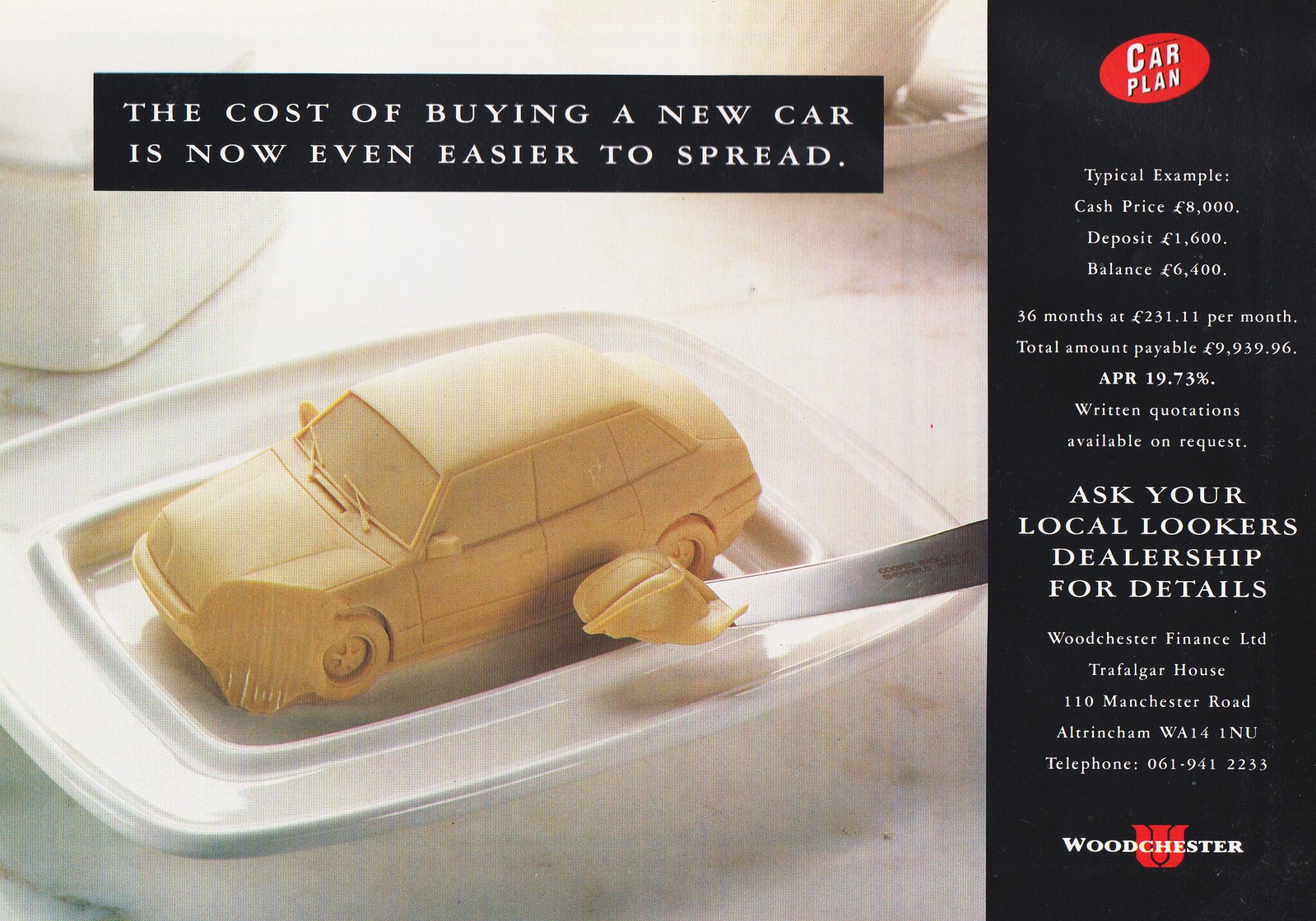This is a detailed advertisement featuring a color photograph set indoors. The centerpiece of the ad is a pat of butter intricately sculpted into the shape of a sedan. The car, cleverly positioned on a small butter dish, has the driver's side headlight and part of the front scooped off by a butter knife which is being held above it. Above the image, a black text box reads, "The cost of buying a new car is now even easier to spread."

On the right side, a black rectangle includes detailed financial information in white text: "Car Plan. Typical example: cash price £8,000, deposit £1,600, balance £6,400. 36 months at £231.11 per month. Total amount payable £9,939.96, APR 19.73%. Written quotation available on request. Ask your local Lookers dealership for details." It provides the contact details for Woodchester Finance LTD, located at Trafalgar House, 110 Manchester Road, Altrincham WA14 1NU, with the telephone number 061-941-2233, and features the Woodchester logo with a red 'W'.